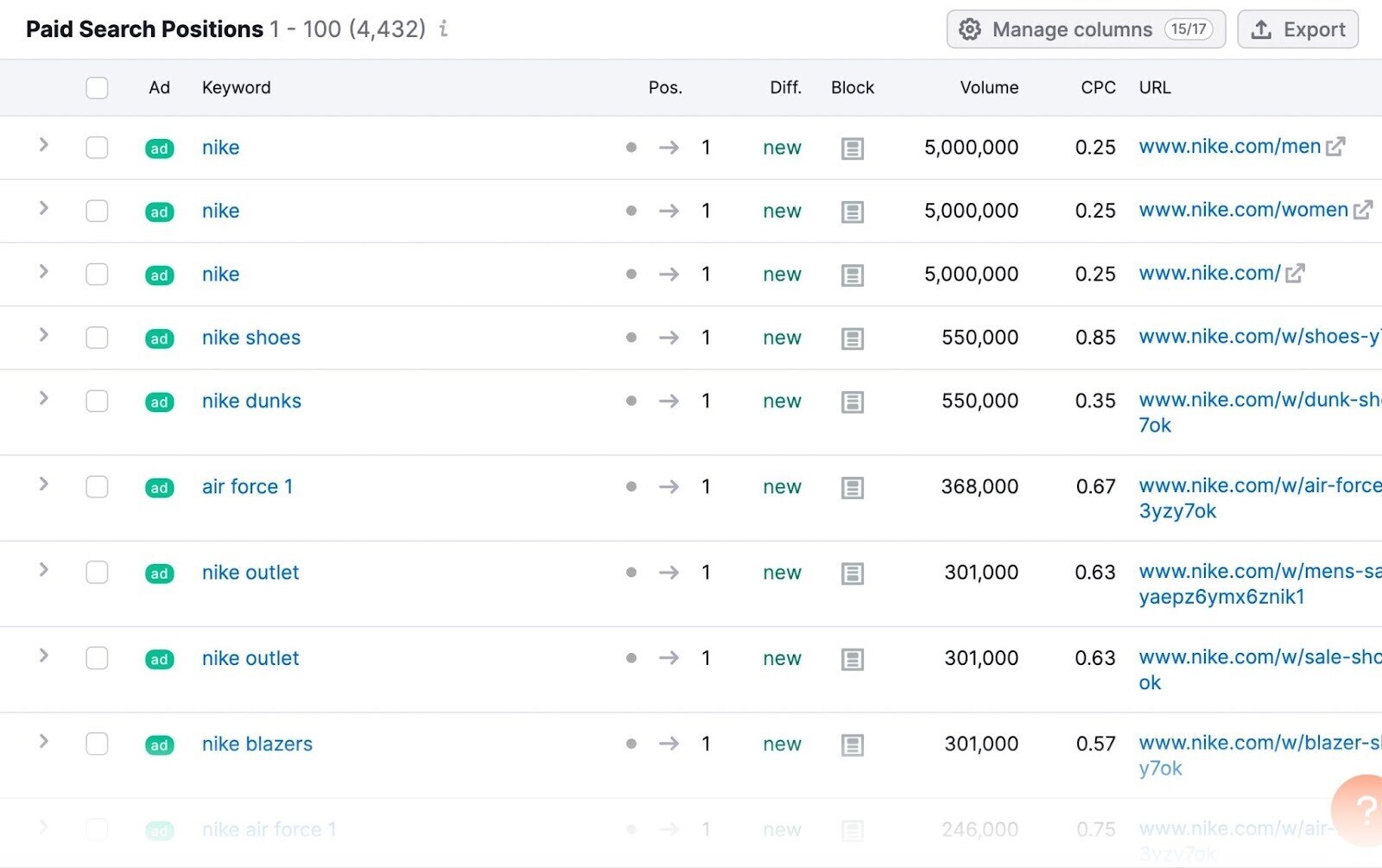The image features a detailed interface, prominently starting with a bold list at the top left labeled "Paid Search Positions, 1 through 100". Accompanying this label is the numeral "4432" followed by a small letter "i" to its right, likely indicating additional information or an info icon.

On the right side of the interface, the section "Managed Columns, 15 of 17" is visible, adjacent to a button labeled "Export". The interface’s top bar includes several interactive elements: a clickable square, an "Add" button, and fields labeled "Keyword", "Block", "Volume", "CPC", and "URL". 

The detailed list begins with an entry showing:
- "Add"
- "Nike"
- An arrow pointing to the right
- The numeral "1"
- The label "New"
- Volume: "5 million"
- CPC: "0.25"
- URL: "www.nike.com/men"

Continuing down the list, there are a total of nine lines, each pertaining to different Nike-related search entries, including "Nike shoes", "Nike Outlet", and "Nike Blazers".